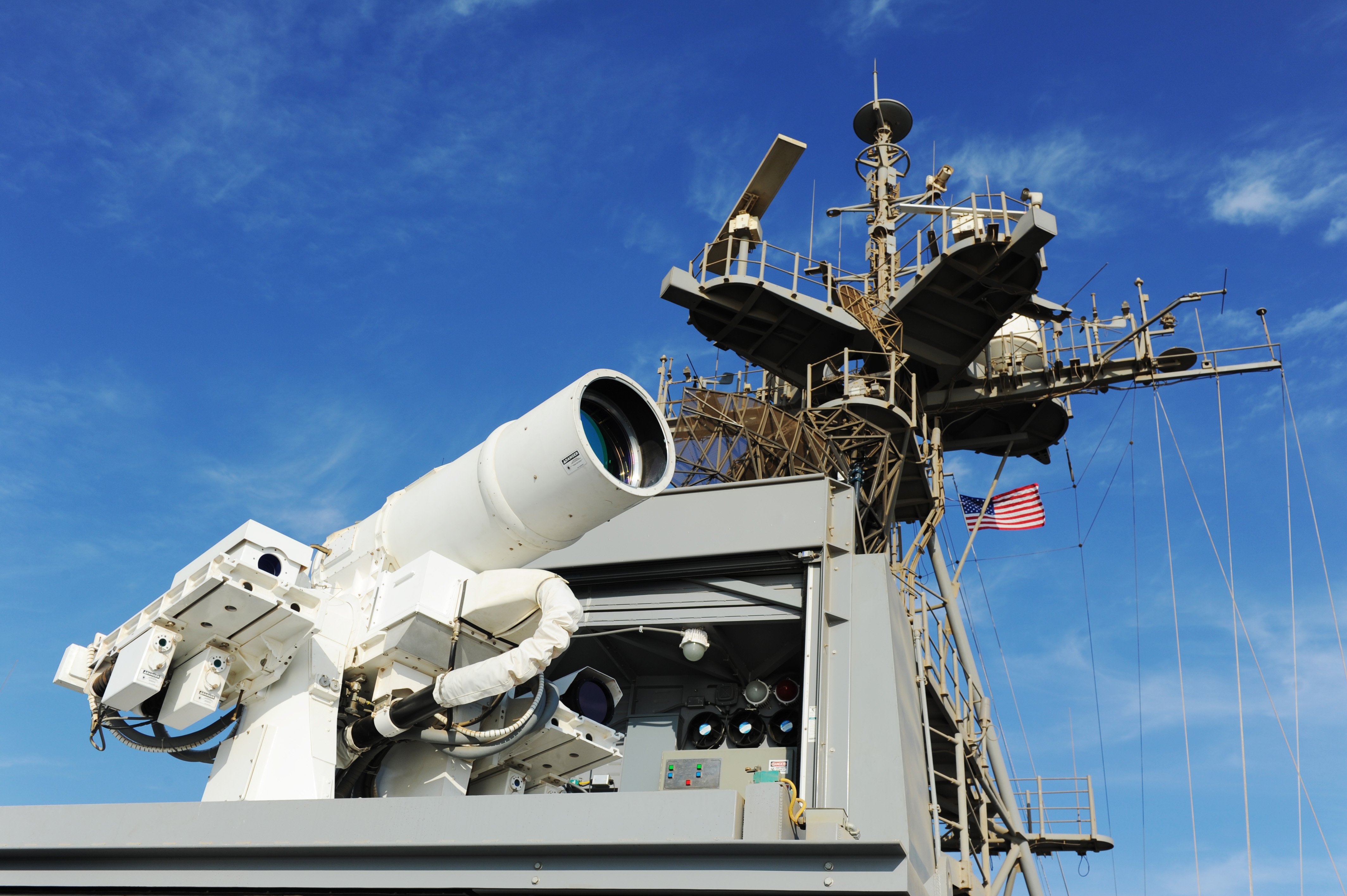The photograph captures a daytime scene taken from the deck of a military ship, identified by its gray paint and the presence of various sophisticated equipment. Dominating the foreground on the left side is a white machine with a tube-like structure, resembling a large telescope or long-range viewfinder, pointed east. This machine is mounted on a gray base adorned with various angular items and cables. Rising above this is a gray tower featuring multiple supporting struts, wires, and what appear to be spinning radar equipment. The tower has several balcony-like sections and is topped with a plus sign-shaped structure. An American flag can be seen blowing in the wind below this uppermost structure. The bright blue sky with wispy clouds forms the backdrop of this detailed maritime scene.